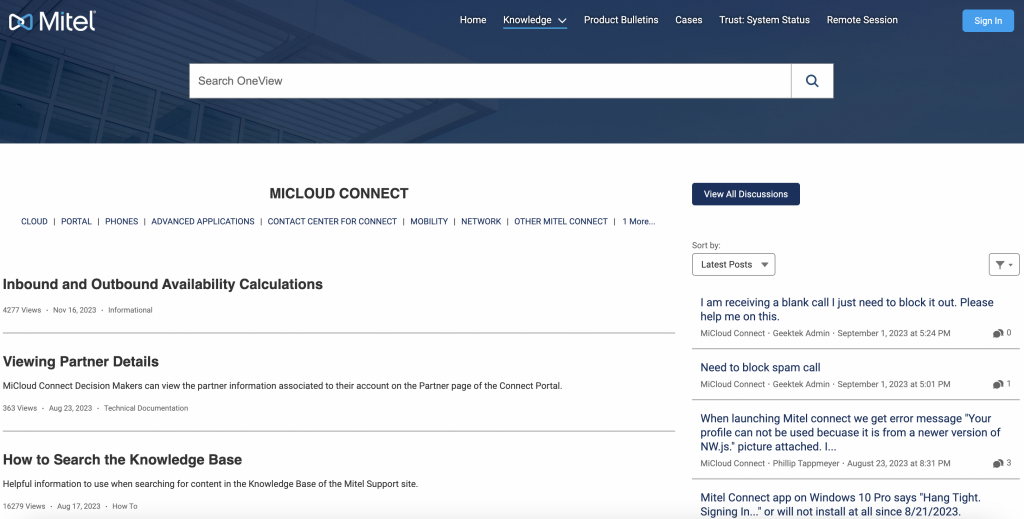This screenshot showcases a page from an application or program named "MITEL." Displayed in the upper left-hand corner, the MITEL logo is situated on a thick blue bar spanning the top of the interface. Adjacent to the logo is a search bar that allows users to enter and search for specific terms. The uppermost section of the page features a horizontal navigation menu, which includes the following headings: Home, Knowledge, Product, Bulletins, Class, Trust, System, Status, and Remote Session. 

On the far right of this menu, there is a light blue "Sign In" button for user authentication. The main section of the page prominently displays the title "McLeod Connect," followed by three detailed subheadings: "Inbound and Outbound," "Availability Calculations," "Viewing Partner Details," and "How to Search the Knowledge Base." The interface appears organized and user-friendly, guiding users to efficiently access various features and information.